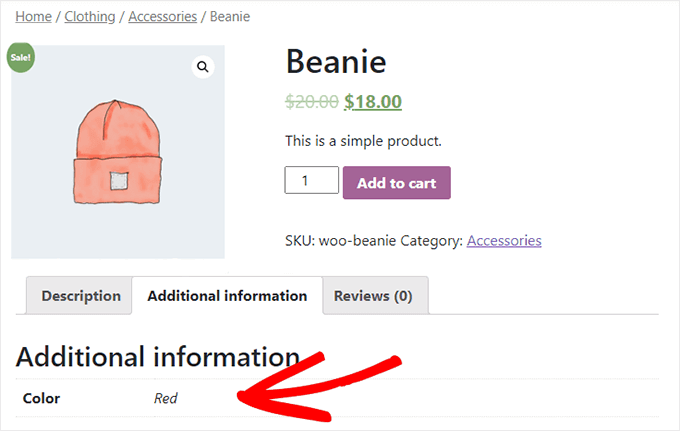The image depicts a webpage from an e-commerce site displaying a product listing for a red beanie. At the top of the page, navigational tags are visible, labeled "Home," "Clothing," "Accessories," and "Beanie." In the main section of the page, the word "Beanie" is prominently displayed, alongside its price which has been reduced from $20 to $18, indicated by the original price being crossed out. 

The beanie is described as a simple product, with a default quantity set to 1, and features a vibrant purple "Add to Cart" button below it. The beanie itself is illustrated, showcased in red with a white tag attached to it. A green sale icon is also present, denoting the item's special discount. 

The webpage is organized into various sections such as "Description," "Additional Information," and "Reviews," the latter of which currently shows zero reviews. The SKU for the beanie is listed as "woo-beanie," and it is categorized under "Accessories." 

At the bottom of the page, under "Additional Information," the color is specified as red in bold text, with an arrow pointing towards this detail. The majority of the webpage features a clean design with a white background and black text, highlighted by occasional gray sections at the top. The image of the beanie stands out against this neutral background, adding a burst of color to the page. Overall, the layout and elements suggest a typical e-commerce platform where users can browse and purchase various products.